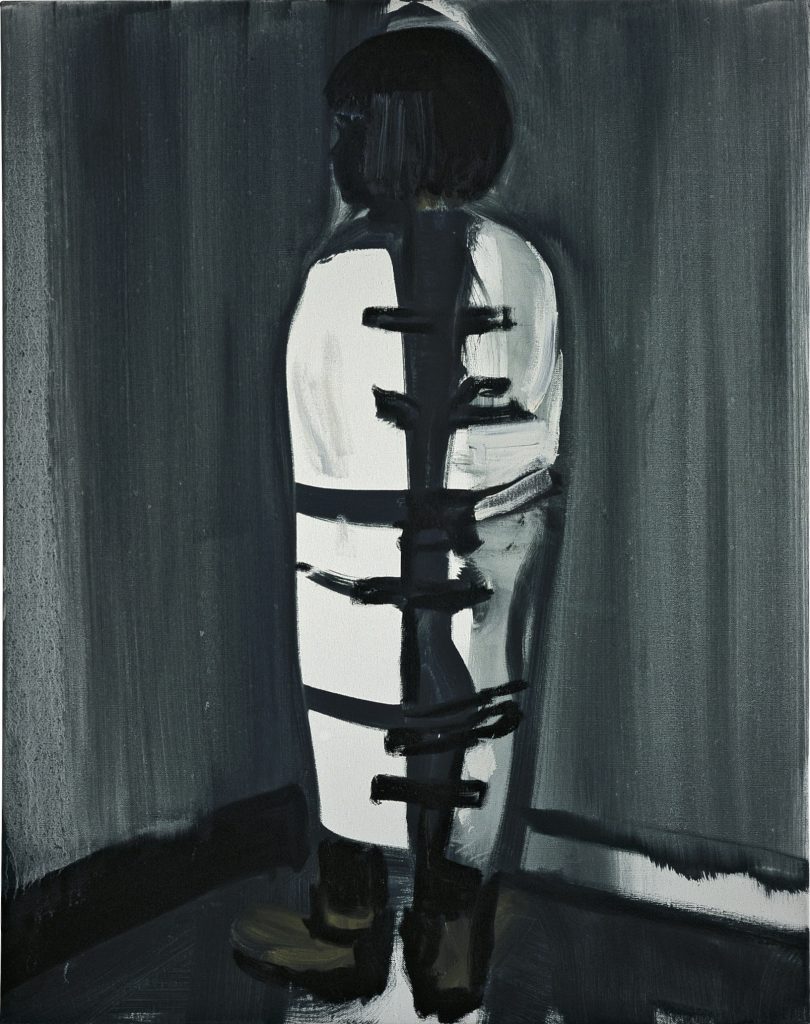The image is a slightly abstract, yet detailed painting of a person, possibly a young woman or child, standing in the corner of a dimly lit room. The painting uses predominantly dark colors, with the exception of the stark white garment the figure is wearing. The background consists of vertical brushstrokes in shades of black and dark gray, representing walls, with a baseboard that alternates in color—white on one side with a black tip, and black on the other side. The nearly black floor adds to the overall dark ambiance.

The individual, depicted from the back, is restrained in a white straitjacket, which is tied up with black strings or buckles running vertically down the back. The figure has short, shoulder-length black hair with bangs, partially turned left, revealing only the blacked-out silhouette of their face. They are wearing brown boots that contrast slightly with their dark attire and the grim setting.